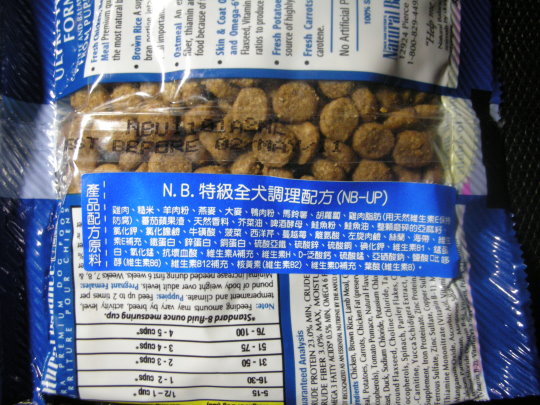This color photograph shows a close-up of the back of a horizontally resting plastic food bag on a black surface, possibly a tabletop. The middle of the bag has a transparent section revealing brown, circular kibble, suggesting it might be pet food. The packaging predominantly features blue and white colors, with various texts both in Chinese and English. The blue rectangle in the center contains Chinese characters, while adjacent sections have English writing and numerical ingredient details like "crude protein 23%", "crude fiber 3%", and specific components such as "omega-3 fatty acids," "chicken brown rice," "lamb meal," "chicken fat," "duck," and "sodium chloride." Upside-down and rotated texts, including a nutritional or serving size label in black on white, further emphasize the package's rotated orientation.